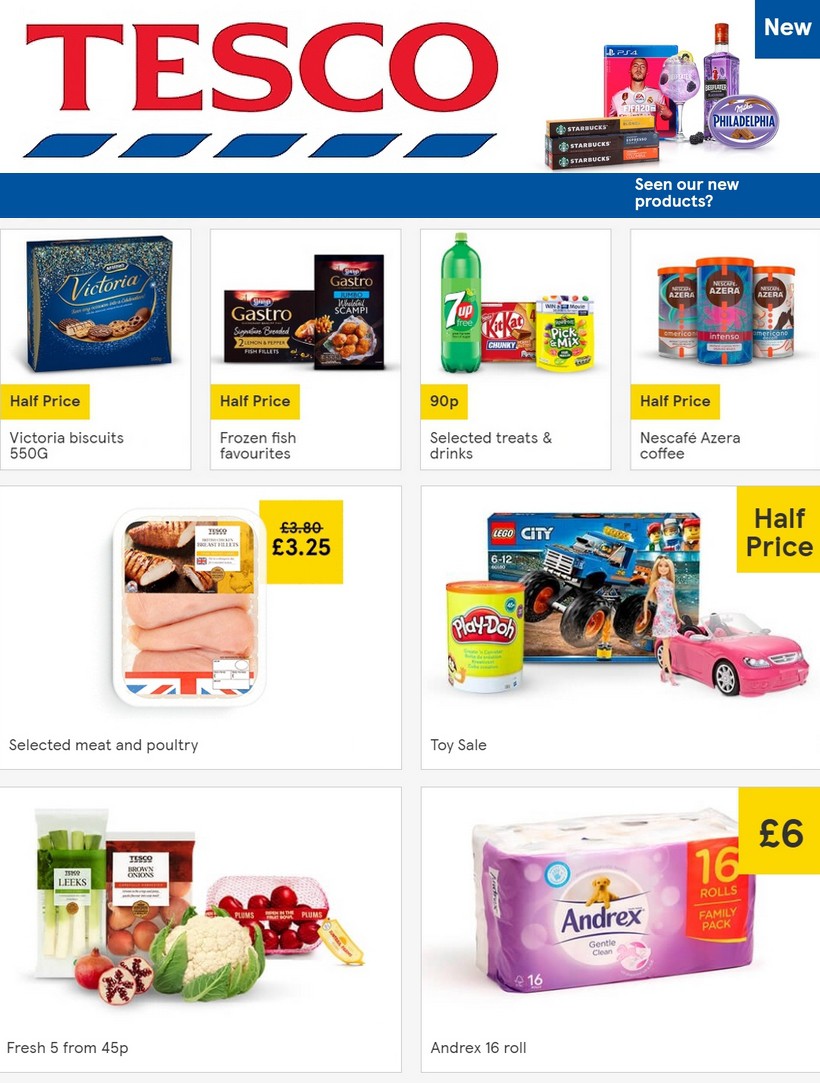This image appears to be an advertisement from a website for Tesco, indicated by the large, bold red "Tesco" at the top. Below the heading, there are five semi-rectangular blue shapes that highlight various new products. Adjacent to them are smaller images including a Starbucks logo, a PS4 game, a bottle of purple liquid, and the Philadelphia brand, marked with "new" in a blue box. Separating these images from the rest of the content is a long rectangular blue box with the text "Seen our new products".

The advertisement showcases three rows of different products. The first row features Victoria biscuits on the left, followed by frozen fish, a bottle of 7Up, KitKat bars, and a pick-a-mix selection. Additionally, there is Nescafe Azera coffee with three containers displayed. The second row is labeled "Selected Meat and Poultry" and includes a picture of chicken. This row also highlights various toys, including Play-Doh, Lego City, and a Barbie car. The final row displays a selection of vegetables – including cabbage, tomatoes, and mushrooms – as well as an image of toilet paper.